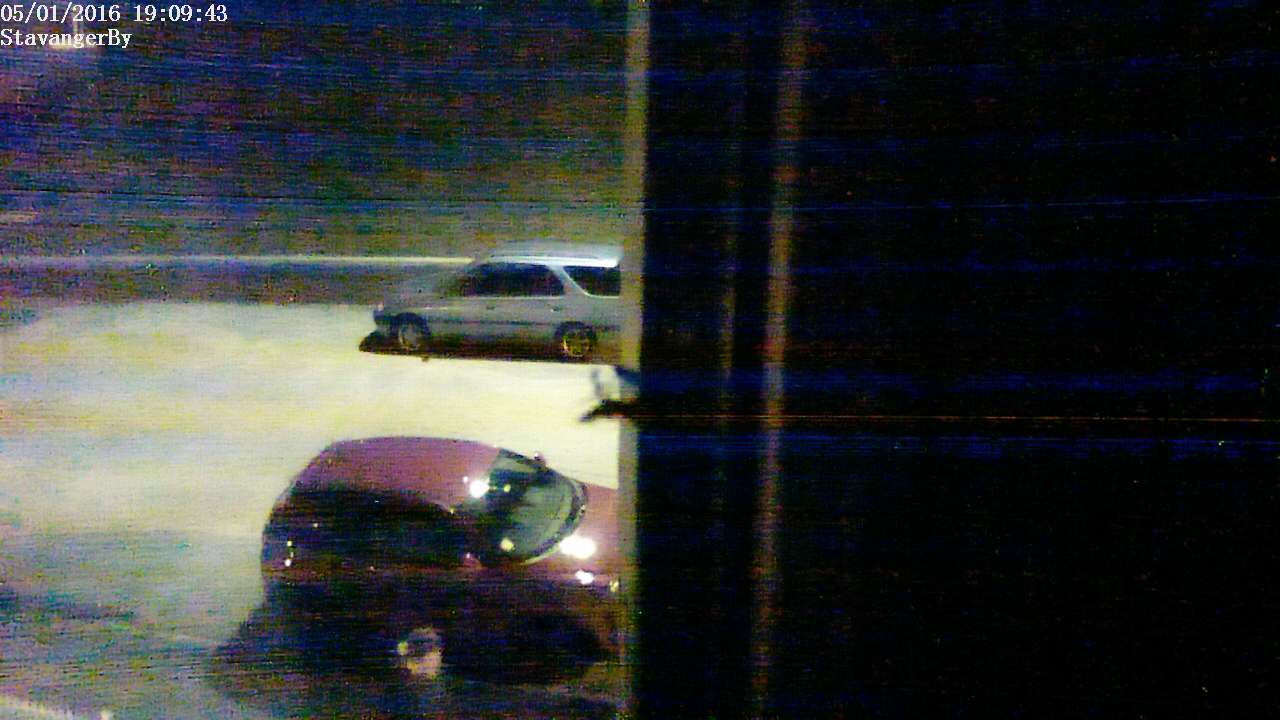In this security camera footage, the camera is positioned within a building, peering out of a window to capture the scene outside. The timestamp on the top left corner reads "05-01-2016 07:09:43," indicating that the image was taken in the early morning hours, despite the surrounding darkness. The words "Stavanger By" are prominently displayed in white letters on the same corner. Illuminated by street lights, the road outside takes on a grayish-yellow hue. The dimly lit scene reveals two cars: a gray one, resembling a Volvo, and a red car with a noticeably darker windshield. There is also a shadow hinting at a third vehicle on the left, though it remains mostly out of frame. The right side of the photograph is dominated by the dark interior wall, suggesting that the camera is slightly off-center and focusing mainly on the outdoor area. The ambient streetlights add a subtle glow to the road, casting shadows and providing limited visibility in this otherwise dark snapshot of the early morning cityscape.